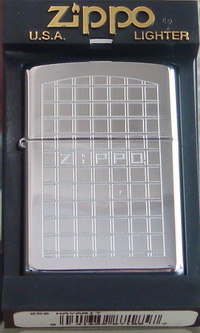The image showcases a Zippo lighter still encased in its original packaging. The packaging is predominately dark blue with silver accents, and prominently features the text "Zippo USA lighter" embossed in gold at the top, where the "I" in "Zippo" is creatively designed as a candle. The center of the packaging houses a silvery section with a checkered pattern of vertical and horizontal lines, within which "Zippo" is also inscribed. The lighter itself, nestled securely in this section, is highly polished and bright silver in color. At the bottom of the packaging, a white sticker with a black barcode is visible, positioned for easy scanning during processing. The overall presentation combines elements of silver, gold, blue, white, and black, encapsulating the classic and sophisticated design of a Zippo lighter.